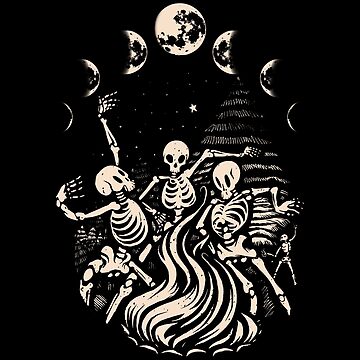In this black-and-white drawing set against a dark, black background, a striking scene unfolds. At the top, an arc displays the phases of the moon, starting from a slender crescent on the left, gradually growing to a full moon at the center, and then diminishing back to a crescent on the right. Below this lunar arc, a stark tree outlined in black and white stands beneath a lone star and several white dots that resemble stars scattered across the night sky.

Dominating the center of the image are three skeletons, dancing animatedly. The skeleton in the middle appears to wear a flowing cape, adding a dynamic element to the scene, while the one on the right gazes upward towards the moon. They dance around what looks like a white fire, its flames encircled by rocks, suggesting a ritualistic gathering. The artist employs strong black outlines and crisp white details to bring the scene to life, creating a mesmerizing and eerie illustration without any accompanying text. The overall effect is both haunting and captivating.